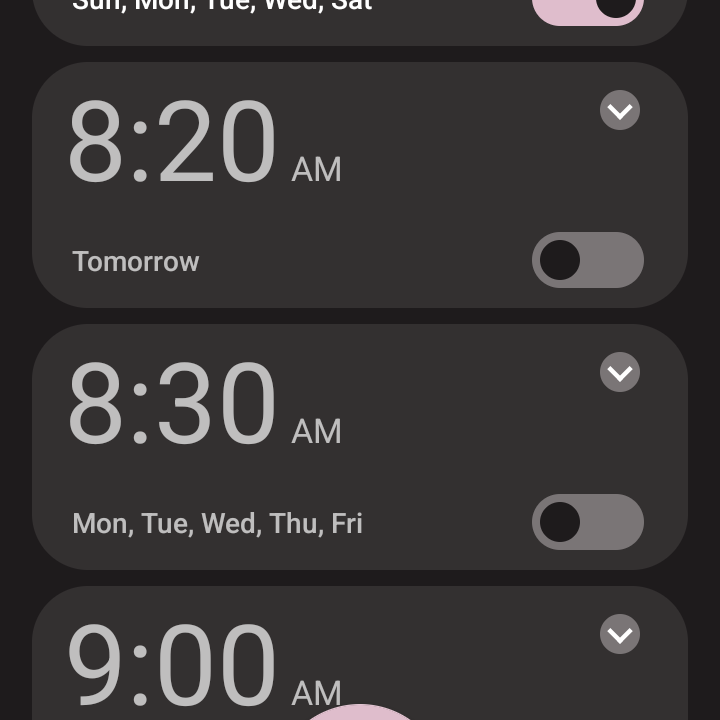Screenshot of a mobile phone displaying an alarm settings interface against a black background with white text. The screen shows multiple alarm configurations:

1. The first alarm is set for 8:20 AM, scheduled for the next day.
2. The second alarm is configured for 8:30 AM, active on Monday, Tuesday, Wednesday, and Friday.
3. At the bottom, an alarm is set for 9:00 AM, but it's unclear whether it is activated.
4. Another alarm is at the top of the list, set for Sunday, Monday, Tuesday, Wednesday, and Saturday, but the specific time is cut off and not visible. 

The screenshot reflects various alarms with some marked as active while others are turned off. A small portion of the surrounding interface is also visible, indicating it might be a tablet or a larger phone screen.